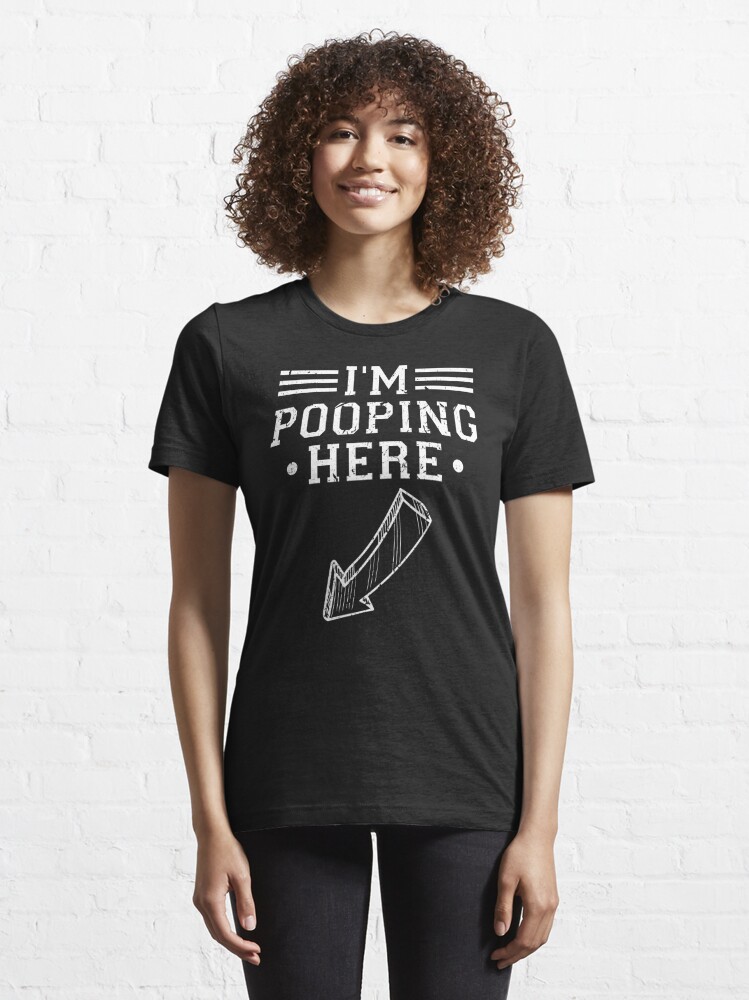In this well-lit, professionally-taken photograph, a light-skinned Black woman with short, curly brown hair that forms a halo around her face is standing against a painted white brick wall. She is smiling at the camera, exuding a humorous and cheerful vibe. She is wearing a short-sleeved black t-shirt with a bold white graphic that reads "I'M POOPING HERE" across three lines of text. The word "I'M" is flanked by three horizontal lines on either side, while the word "HERE" is accented by a white dot on the left and right sides. An arrow points from the text towards her side near her stomach. She pairs the t-shirt with dark-colored leggings, and her arms hang naturally by her sides. The photograph is minimalistic, featuring no additional colors or text beyond those described, and captures the engaging and playful nature of the t-shirt's design.